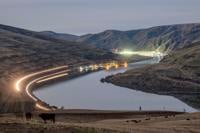This small, detailed photograph captures a serene dusk scene set in nature. Situated in a canyon, a blue river meanders through the center of the image, flanked by rising mountains on either side. The mountains display average vegetation, adding a natural charm to the landscape. In the foreground, a flat expanse of grayish-brown dirt distributes itself over the lower portion, with two tiny cows distinguishable on the lower left while small, black specks on the right suggest the presence of more distant animals.

The left riverbank is adorned with a long row of yellow lights that follow the river's curve, possibly illuminating man-made structures like a factory, buildings, or a dam. Additional bright white lighting is seen farther off in the background, hinting at another structure nestled between the encompassing mountains.

Off to the right side of the image, the mountainous landscape continues, with an occasional spotting of tiny, ant-sized people walking in front of the water. The sky above is a combination of dark gray and clear blue, with minimal cloud coverage, occupying about one-fifth of the image at the top and spanning from left to right. This scenic photograph beautifully melds the serene elements of nature with subtle traces of human presence.